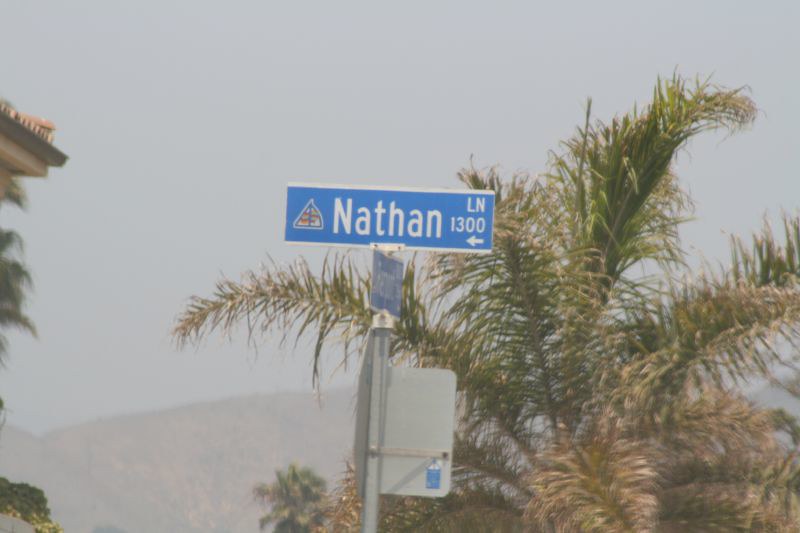A foggy day in a warm climate is captured in this photograph. The scene is shrouded in a dense gray fog that partially obscures the rolling hills in the background on the right side. The upper right corner of the image features part of a building with some greenery peeking through, adding a touch of life to the muted palette. Dominating the left side of the frame, a full palm tree stands tall behind a street sign. The sign, elevated on a silver pole, is blue with white trim, indicating "Nathan Lane, 1300" and includes an arrow pointing to the left. The composition suggests an ordinary locale named after the celebrity Nathan Lane, adding a hint of intrigue to the otherwise serene and misty atmosphere.